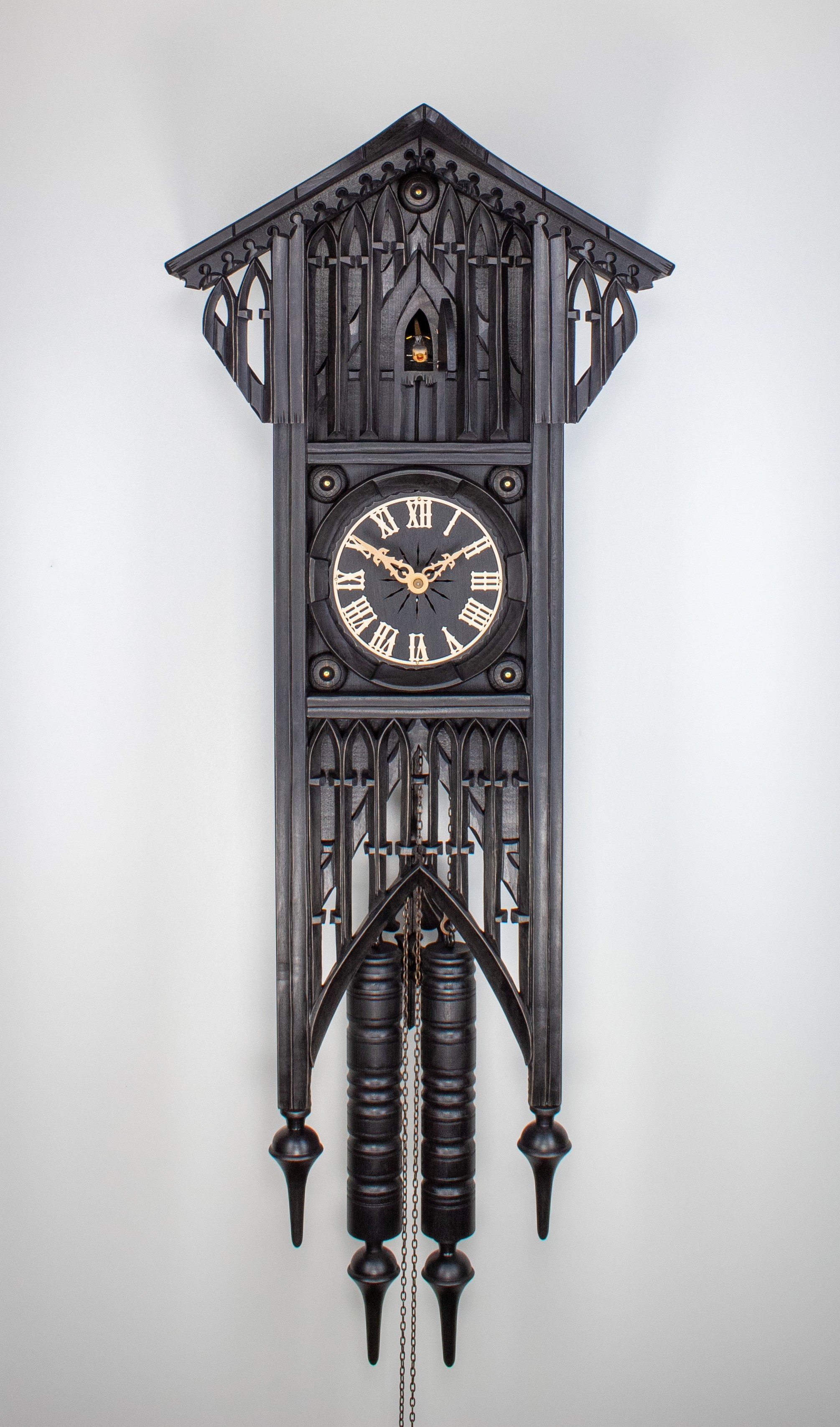This is a photo of a long, vertically aligned, European-style wall clock set against a light gray background. The clock is predominantly black, creating a striking contrast with its gold-colored accents. The clock's design features a triangular, roof-like tip at the top, which includes a tiny doorway. Here, instead of a traditional cuckoo bird, there is a small figure, possibly holding a drum. The clock face in the center is dark gray and displays gold Roman numerals alongside gold minute and hour hands, adding a touch of elegance.

The structure of the clock is a vertical rectangle that extends downwards, culminating in spire-like tips at the bottom corners. Suspended from these corners are two chain-like rods, each ending with metal or wood knobs, likely essential for the clock's movement. This decorative wall clock stands out as a detailed and intricate piece, combining functional and ornamental elements.